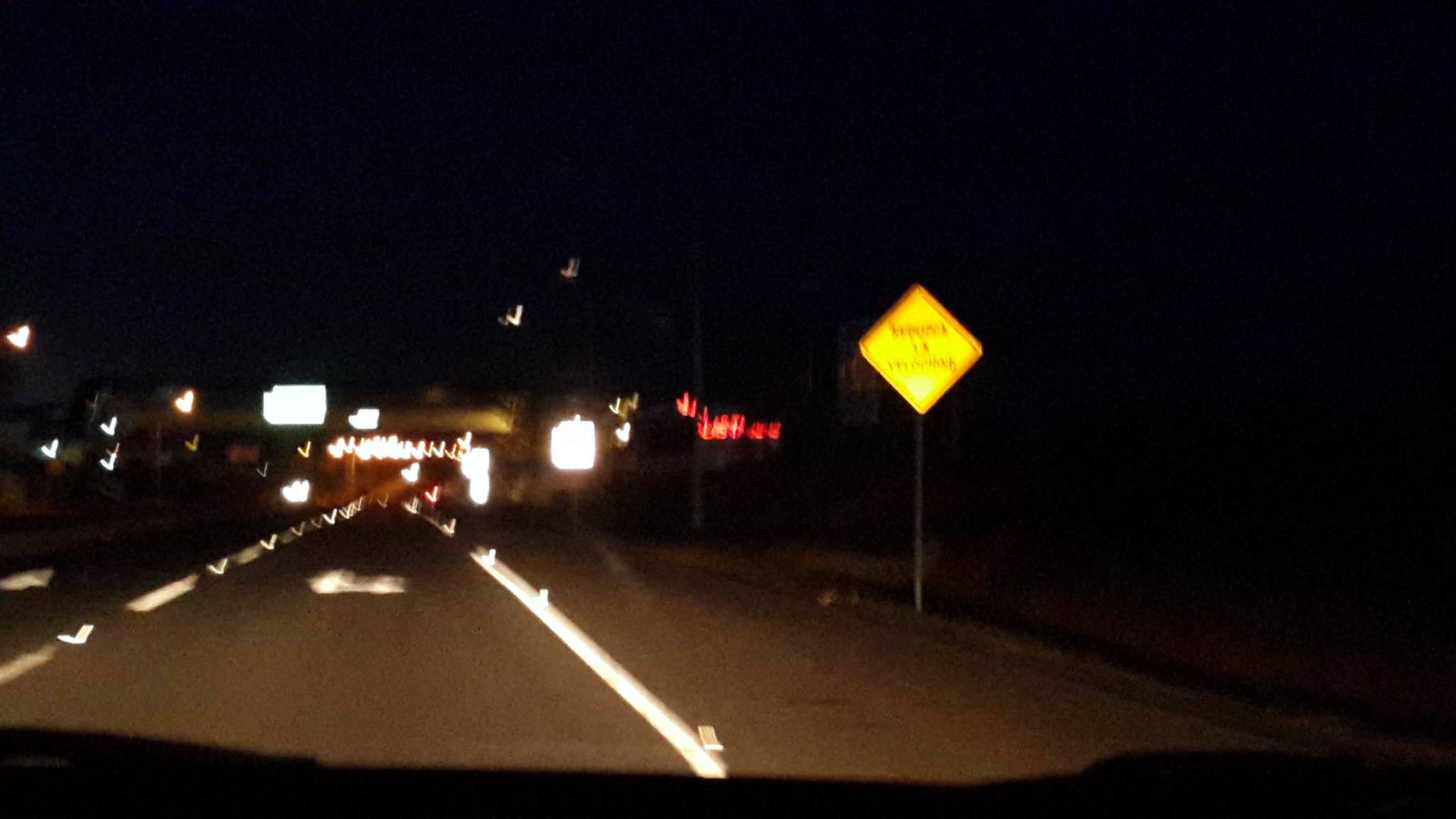A nighttime photograph captures the view from inside a vehicle, partially revealing a blurry and grainy black dashboard at the bottom of the image. The road ahead is illuminated by the vehicle's headlights, displaying the dark pavement with white reflective lane markings. A golden-black road sign stands prominently to the side, and more reflective road signs are visible in the distance. Red taillights of vehicles ahead and white headlights of oncoming traffic dot the parallel lanes. The super far background hints at distant white city lights under a pitch-black sky. An overpass spans the roadway overhead, while light poles can be seen faintly in the distance. On one side of the road, some grass patches are visible. Arrow markings on the road surface further guide the way.